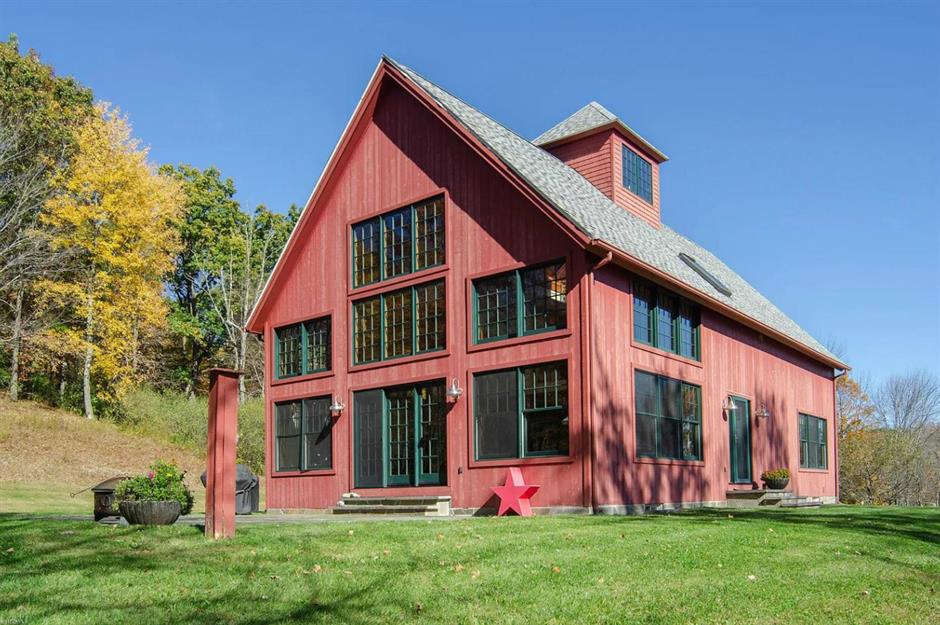This image captures an outdoor scene featuring a large, two to three-story red wooden house, possibly used as a retreat. It has a distinct light-colored, arch-shaped roof with a skylight. The house is characterized by its green-framed windows, which include multiple small panes, and a prominent green door. There's a front entrance with a couple of steps leading up to it, flanked by two lamps. Beside this entrance, there's a potted plant and some stone planters holding green shrubs.

In front of the house, there's a small paved patio and a well-manicured lawn. Additionally, a noticeable red star sculpture leans against the front of the house, near one of the windows. The house also features a side door accessible via two steps. Surrounding the house are numerous trees, some with green leaves, others bare or with yellow leaves, casting large shadows on the building. The sky is blue, suggesting it's late in the evening, and the overall setting hints at a tranquil, retreat-like atmosphere.